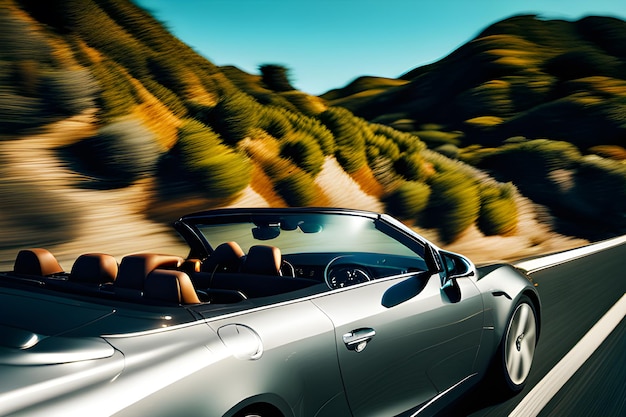The image appears to be an AI-generated high-speed photograph of a steel gray convertible sports car, almost silver in hue, traveling down a highway on the left side of a solid white center line. The car displays numerous anomalies suggestive of digital manipulation, including multiple, oddly spaced headrests and duplicated rear and side view mirrors. The front seats feature one missing passenger headrest and two headrests on the driver’s side. The car’s interior is a striking brownish-red leather. The background showcases a blurred hillside in rust and tan with green bushes, and another hill further back with brown, tan, and gray splotches. The bright turquoise sky contrasts with the digitally distorted landscape. Notably, the road, seen clearly beneath the front right wheel, has no yellow stripe, only white lines bordering the narrow lane, enhancing the otherworldly feel of the image.